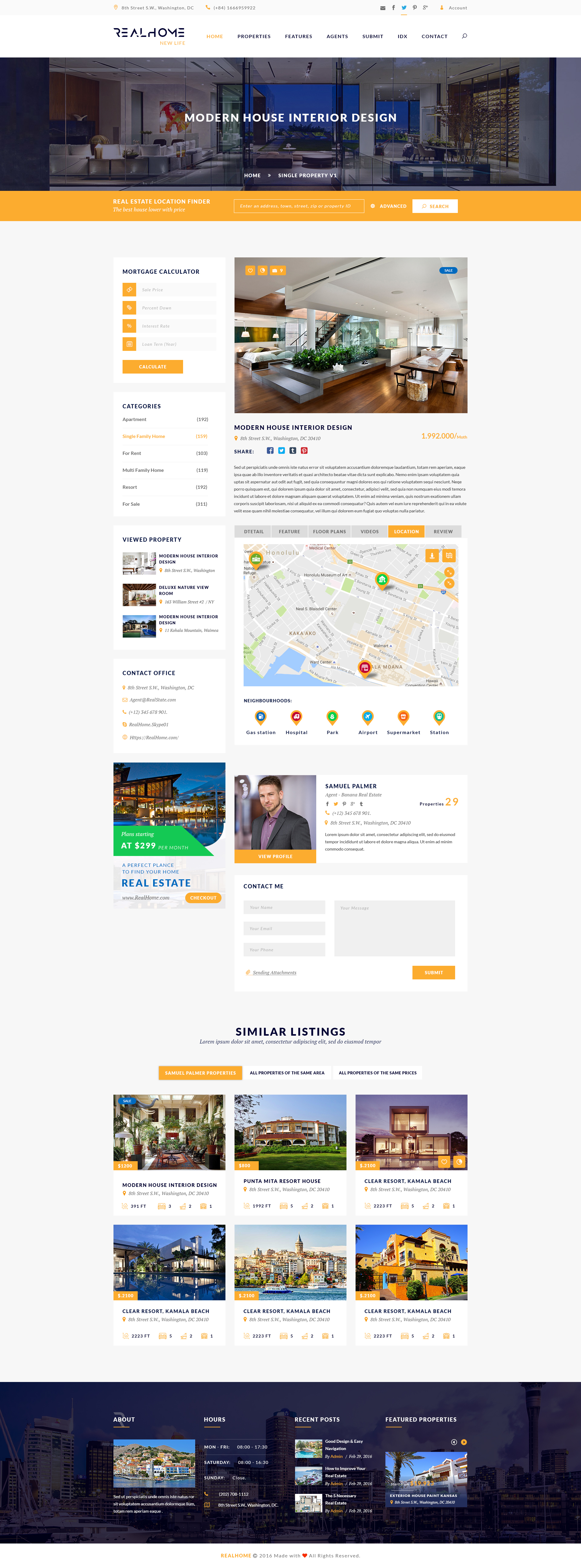This vertical rectangular image features several distinct elements organized in a structured format:

1. **Top Section**: The image begins with black font at the top, though the text is quite small and difficult to read.
   
2. **Main Image Overlayed with Text**: Below the top text is a horizontal image that spans the width of the frame. This image is somewhat indistinct, but it is overlaid with large, white, all-caps text that reads "MODERN HOUSE INTERIOR DESIGN," suggesting that the underlying image likely depicts a contemporary home interior.

3. **Gold/Yellow Rectangle**: Beneath the main image is a gold or yellow rectangular box that runs horizontally across the image. This box contains small white lettering, which is hard to distinguish.

4. **White and Yellow Horizontal Text Box**: Towards the right-hand side of the gold/yellow box, there is a white horizontal rectangle with tiny yellow text within it, making the content difficult to decipher.

5. **Detailed Data Visualization**:
   - On the left side of this lower section is a vertical rectangular image featuring a graph with black text. The graph itself consists of yellow bars and additional lines indicating further data points.
   - Adjacent to the graph is another image, followed by a section of tabulated data and a map.
   - Below the map is a picture of a man with what appears to be accompanying biographical or informational text, though the specifics are unclear.

6. **Central Heading and Listings**: In the center of the bottom third of the image is a bold black heading that reads "SIMILAR LISTINGS."
   - Below this heading are two rows of three listings each, totaling six listings. Each listing includes an image of a home with information provided underneath.

7. **Bottom Section with Background Layer**: At the very bottom of the image is a dark rectangular box. Behind it, partially visible, are images of homes. Superimposed over this background layer are several vertical rectangular boxes, adding another layer of information or imagery.

The composite arrangement of textual and graphical elements in this image suggests it is a detailed real estate listing or a layout within a property magazine.